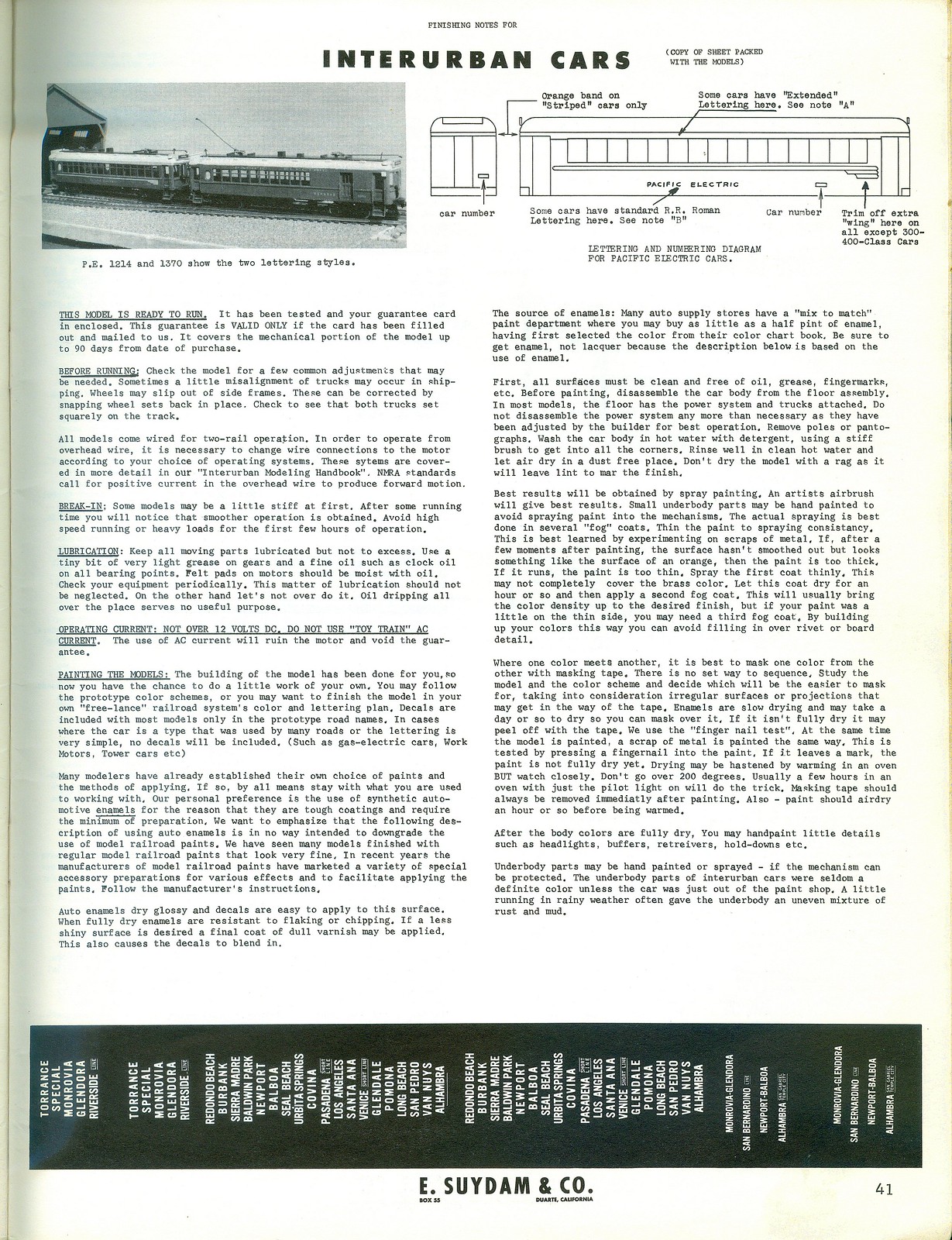The image depicts a printed document in black and white, likely a page from a book or magazine, titled "Interurban Cars." In the upper left corner, there is a black and white photograph of a two-compartment train, characterized by a white top and a dark-colored body, emerging from a triangular roof structure on the left side of the image. Adjacent to this photograph on the upper right is a detailed diagram labeling various parts of the train car. Below these images are two columns of very small font text, each containing several paragraphs. At the bottom of the page, there is a black rectangular section with numerous words written vertically and the name "E. Sudam & Co." located at the very bottom, possibly indicating the company responsible for the document. Additionally, the page number 41 suggests that this is part of a larger publication.